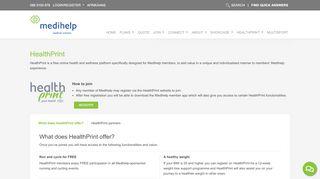**SEO Metahelp App Interface Screenshot Description**

This is an enlarged screenshot purportedly showcasing the interface of the Metahelp app or webpage. The image is horizontally oriented, with a rectangular shape typical of a digital screenshot. At the very top of the screenshot, there is a dark gray border, populated with some text on both the left and right sides. The exact nature of this text is unclear due to the zoomed-in view, but it might include elements such as dates, a search box, or navigational indicators, rendered in a light gray or white font.

Directly beneath this top border, on the left side, the logo and name of "Metahelp" are distinctly visible. The "Metahelp" name is written in a blue font, while the accompanying logo consists of a green, circular design. Adjacent to the logo, on the right, there is a menu bar. The details of the menu options are indecipherable in the zoomed-in view, but it appears to contain around 10 clickable options, forming a horizontal white section against the gray backdrop.

Below the menu, the interface appears to transition to another textual section, also gray, which may serve as a header or descriptive text area. The words "health print" are discernible in this region, suggesting a focus on health-related services or information. There are a few bullet points, indicating the reiteration or summarization of key features or benefits. Among these bullet points, a green button stands out against the gray background.

Further down, the layout includes a prominent white text box labeled "What does health print offer?" This section likely provides detailed information on the services or features of Health Print, as evidenced by the presence of multiple paragraphs of text. The screenshot ends shortly after this descriptive text box, indicating that this section may form the conclusion of the viewed page.